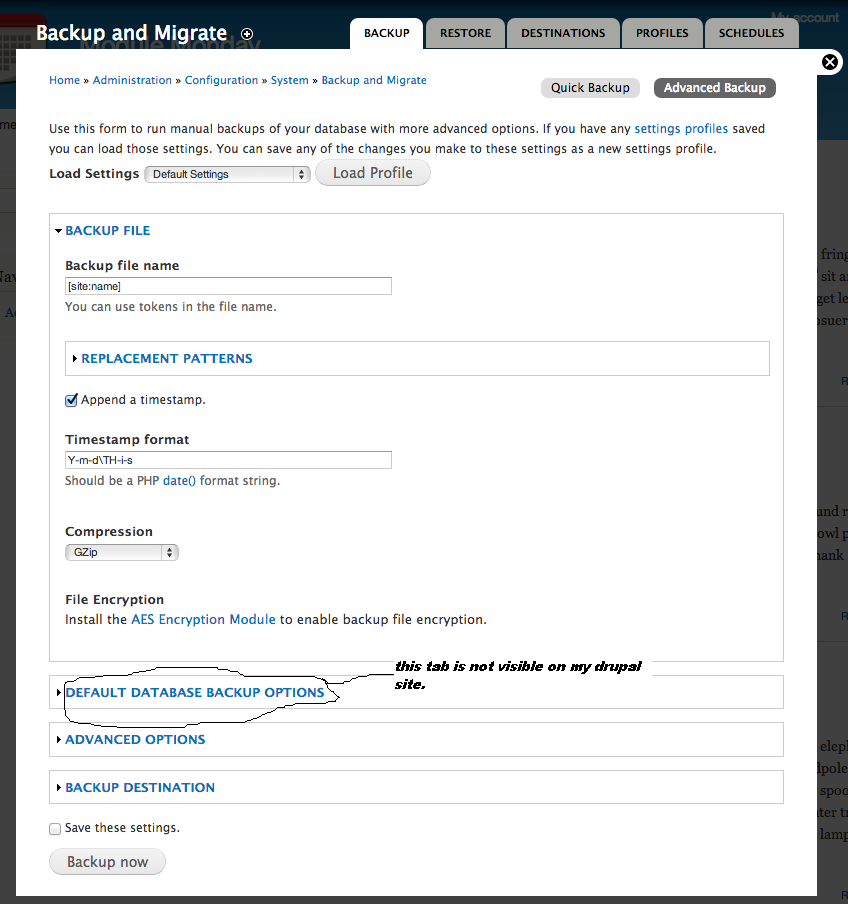The webpage displayed is a vertically arranged, white rectangular interface. At the very top, a black ribbon highlights the title "Backup and Migrate" in white text situated in the top-left corner. To the right, a series of tabs labeled "Backup," "Store," "Destinations," "Profiles," and "Schedules" are arranged in gray with black text. The "Backup" tab is distinctively selected, shown as black text on a white background.

Beneath this ribbon, the page is predominantly white. At the top of this section, a line of bright blue, tiny text reads "Home," "Administration," "Configuration," "System," and "Backup and Migrate." Adjacent to these labels are options for "Quick Backup" and "Advanced Backup."

Below these headings, a gray text block provides instructions: "Use this form to run manual backups of your database with more advanced options. If you have any settings profiles saved, you can load those settings. You can save any of the changes you make to these settings as a new settings profile."

Further down, in black text, it says "Load settings," accompanied by a drop-down menu and a button labeled "Load Profile" to the right. Following this, in bright blue text, the label "Backup file" appears above a box for entering the backup file name. Beneath this, another bright blue label reads "Replacement patterns," with a checked box indicating "append a timestamp." Adjacent to this is another selection box for timestamp format.

Continuing down, a drop-down menu offers compression options. Beneath this, it reads "File encryption," along with the message, "Install the AES encryption module to enable backup file encryption." Additional informative sections extend further down the page, providing detailed backup and migrate functionalities.